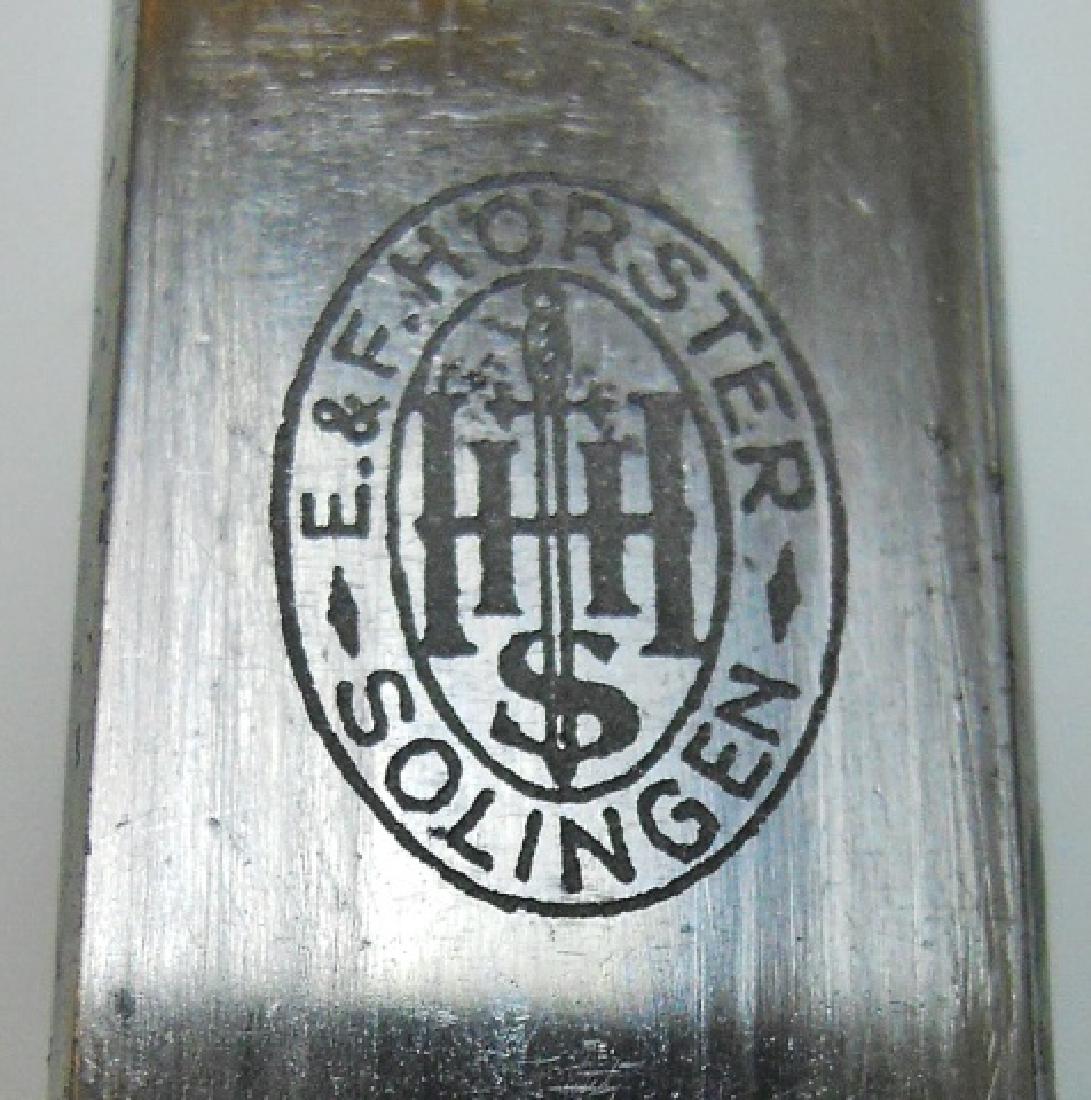In this detailed color photograph, a close-up captures an emblem on a piece of silver metal, which appears weathered with slight scratches and signs of aging, including a hint of rust in the upper left corner. The setting is against a grayish-white background that might be part of a table or wall. The emblem, possibly the logo of a company, prominently displays "E&F Horster" at the top in an arch shape, and "Solingen" at the bottom, all encased within an ovular boundary. Central to the emblem is a downward-pointing sword that intersects with an 'S' at the bottom. Flanking the sword are the letters 'H' on each side, forming a symmetrical design with an 'H' in the middle and another 'H' extending from each side, giving the impression of the sword slicing through an elongated 'S'. The background wood exhibits a vertical grain and adds a rustic texture to the overall metallic aesthetic.